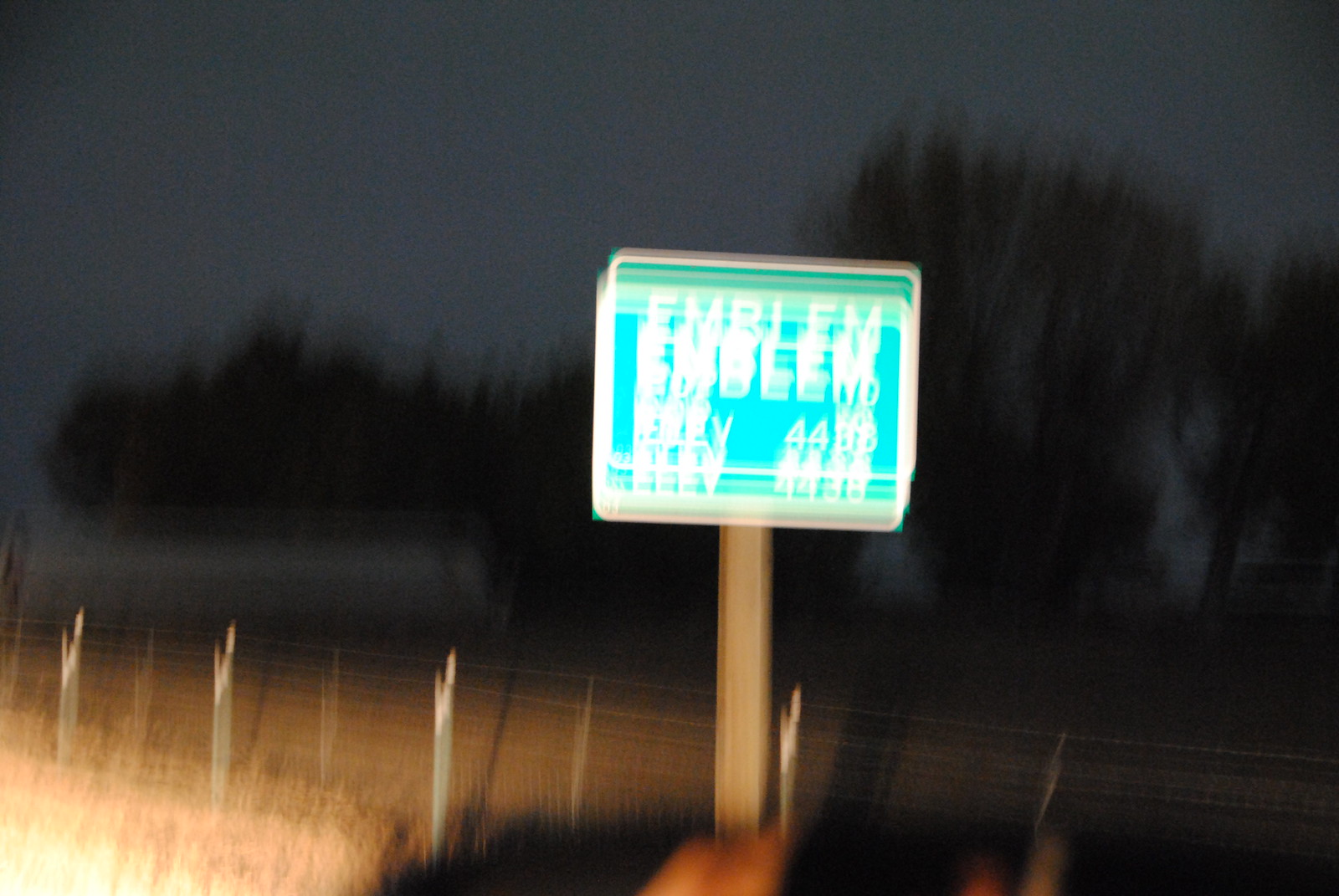This is an extremely blurry photograph taken at night, capturing a green road sign with a white border and white text. The sign is mounted on a light brown post and prominently reads "EMBLEM" at the top, although the rest of the text indicating elevation—possibly "Elevation 4,004" or "4,488"—is smudged and difficult to decipher due to the camera's movement. Behind the sign, there is a wire or chain-link fence, and beyond the fence lies a field of dry, brown grass with shadowy trees. The scene is illuminated primarily by car headlights, casting a bright glare on the sign and the foreground grass. The night sky appears dark blue to gray, adding to the overall dim and shadowy atmosphere of the image.